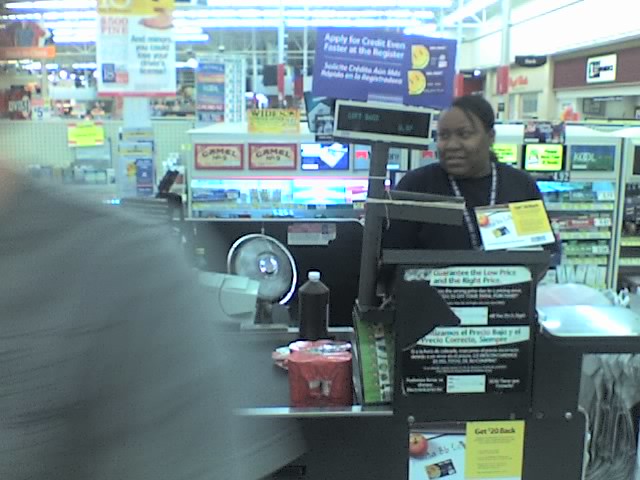This photo captures the bustling scene of a convenience store, likely taken from a low-quality surveillance video. At the center of the image, a cheerful female cashier with dark black skin and hair stands behind a cash register and a conveyor belt, which holds various items, including red cans and a brown bottle. She is dressed in a black shirt and wears a lanyard around her neck, possibly holding a key. Behind her, tall shelves are stocked with cigarette packs and tobacco advertisements, while bright white-blue lights illuminate the ceiling of the spacious store. To the right of the frame, the blurred shoulder of a person in a gray shirt is visible. Additionally, the store features glass display cases and blue and white signs, hinting at the presence of gas tanks outside.